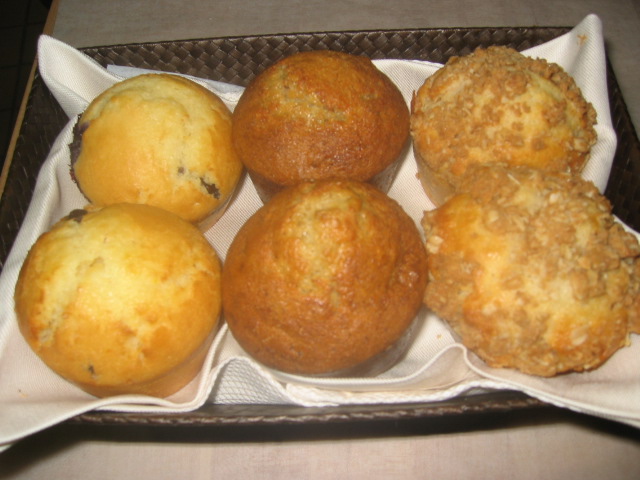In the image, we see a close-up, slightly downward view of a small dark brown woven basket lined with a white cloth or napkin. Nestled inside are six muffins arranged in three rows of two. The muffins vary in color and texture: 

- The top left pair is a golden-yellow-brown, possibly blueberry given the presence of dark blue dots.
- The middle pair appears golden-brown without visible toppings, potentially banana nut muffins based on their color.
- The right-hand pair is a lighter yellow, generously topped with a brown seasoning or crumbly substance, suggesting they might be cinnamon-flavored.

The basket rests on a light gray table, providing a subtle background contrast to the vibrant display of muffins.